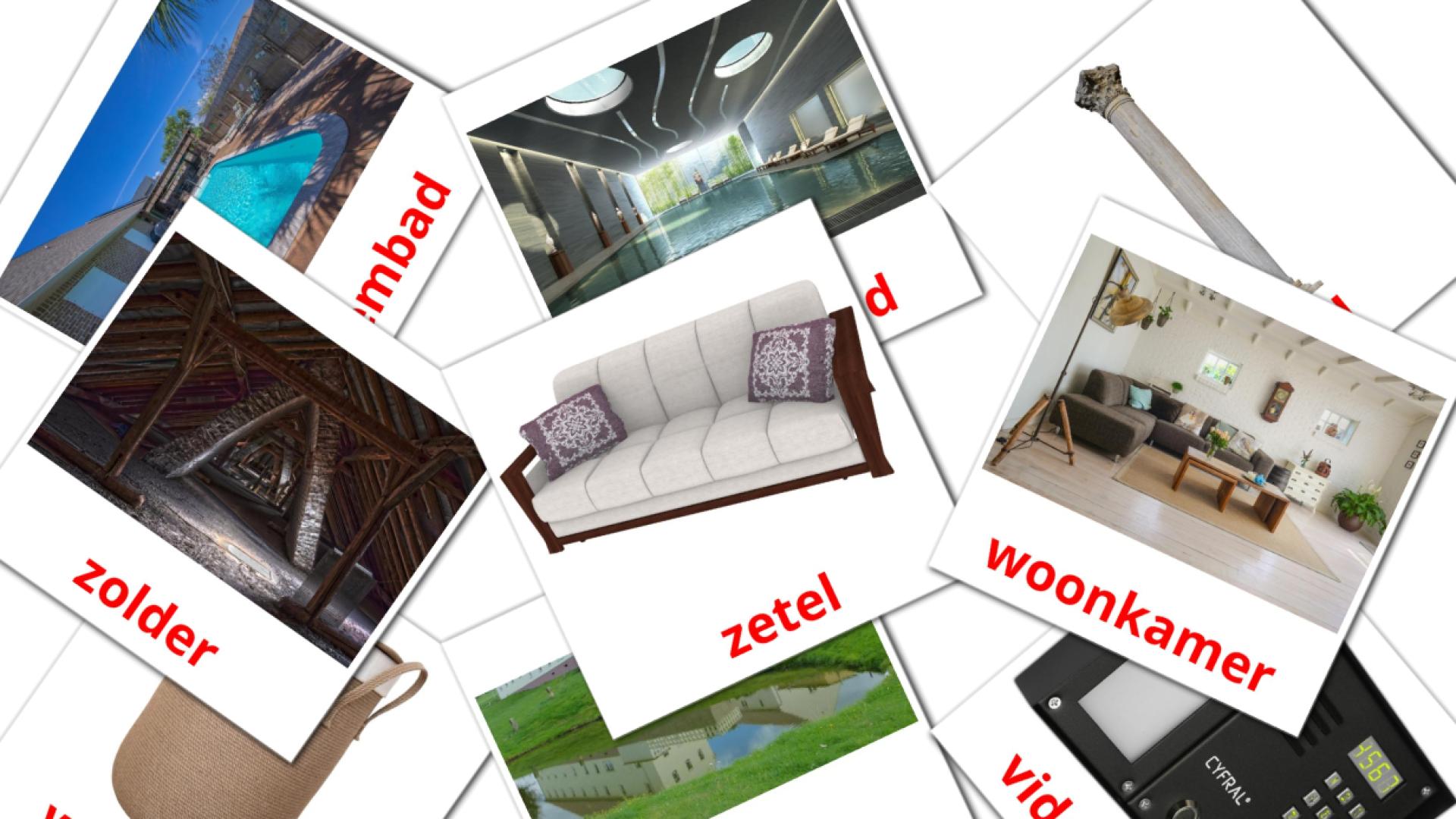The image is a collage on a white background resembling a collection of overlapping Polaroid pictures, which may be computer-generated. Each picture has a red title in the white space below the photograph. 

In the upper left-hand corner, a slightly slanted image shows an outdoor pool, partially covered by another slanted image of a dark, triangular wooden structure labeled "ZOLDER." Centrally, there is a white sofa with gray and white pillows, labeled "ZETEL." Toward the center-right, a living room scene with sofas and additional furniture is labeled "WOONKAMER." Other partially visible images include an indoor pool, an outdoor building with surrounding grass, a tall statue, and a black electronic device, possibly a calculator, with only "VID" visible in the red letters. Additional images depict a large green field, a concrete pillar, and perhaps a tan bag among them.